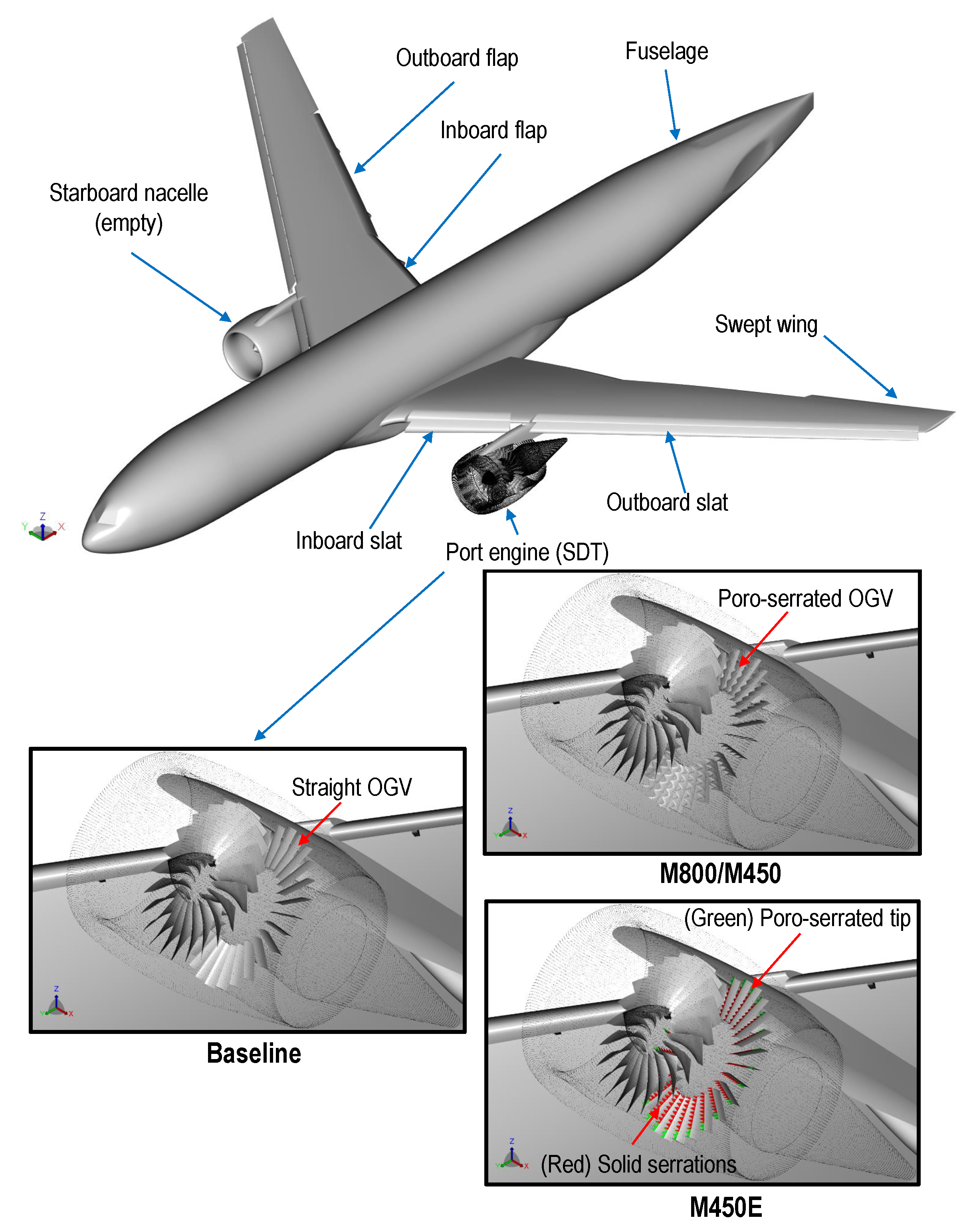This image showcases a detailed diagram of a gray, outlined airplane, illustrating various parts of its structure and different engine components. The plane's key sections are labeled with blue arrows and black text, detailing components such as the fuselage, starboard nacelle, port engine (SDT), swept wing, inboard slat, outboard slat, inboard flap, and outboard flap. Each part is clearly identified with attention to the position and symmetry of the aircraft.

Beneath the diagram of the airplane, there are three close-up rectangle illustrations focusing on engine variations. The first rectangle on the left is labeled "Baseline" and highlights a straight OGV (Outlet Guide Vane). The middle rectangle showcases an engine labeled "M800/M450," featuring a porous serrated OGV, which indicates rougher blade edges for noise reduction or performance enhancement. The last rectangle on the right, marked "M450E," displays a porous serrated tip with distinct red and green highlighting on the components, which likely emphasizes differences in design or material usage. The entire illustration is set against a white background, providing a clear and uncluttered view of both the airplane structure and the intricate details of the engine designs.